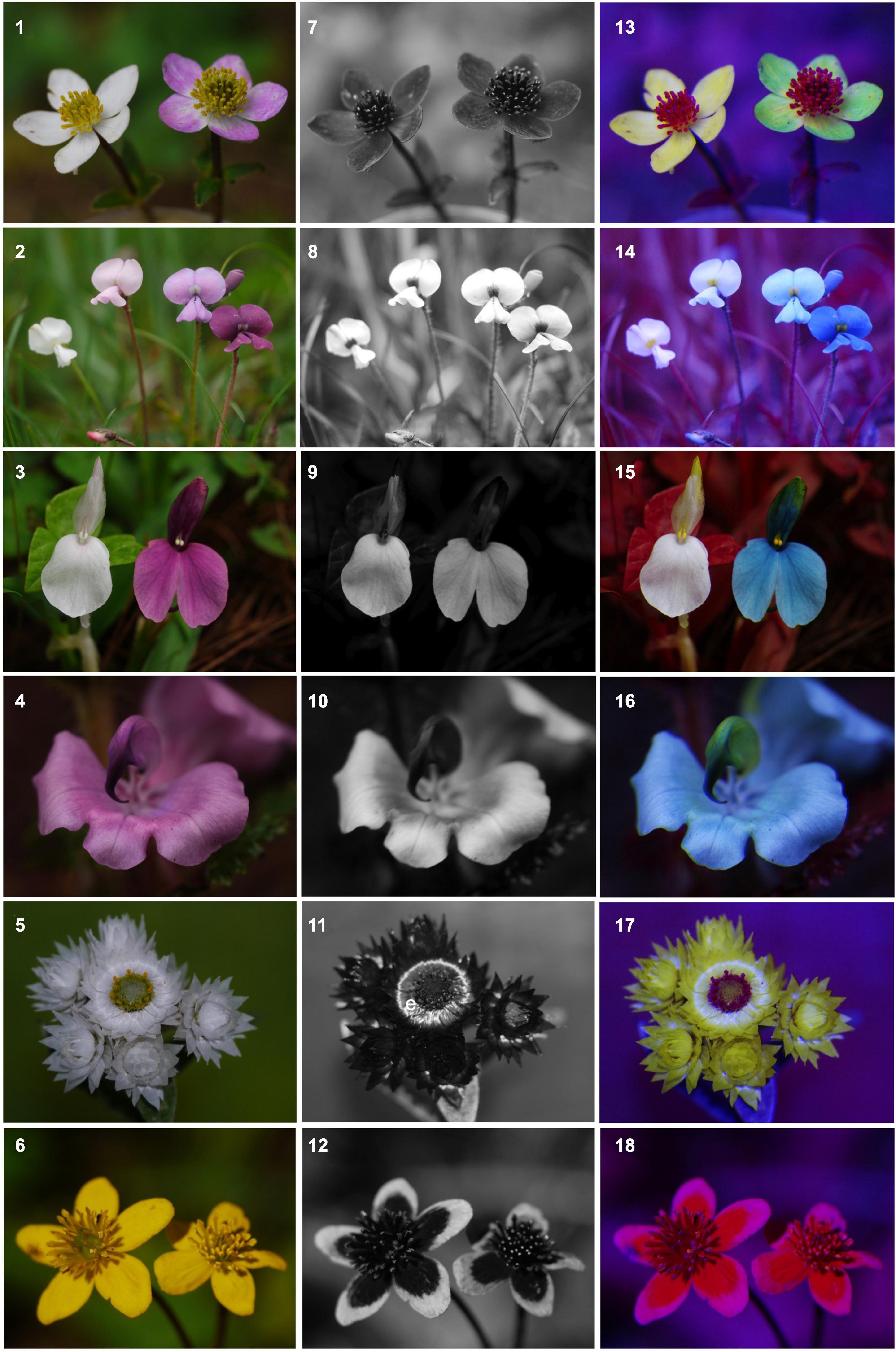The image displays a grid of 18 rectangles, arranged into six rows and three columns, each showcasing photos of various flowers in varying visual styles. The first column presents regular color photos, the second column features the same images in black and white, and the third column highlights the photos with enhanced or reversed colors, possibly resembling UV lighting. 

- **Top Row**: Features two flowers, each with five petals—one white and the other pink—with yellow centers.
- **Second Row**: Consists of four flowers in different shades of pink, each having a rounded shape with a distinctive bottom petal.
- **Third Row**: Displays two flowers side-by-side, each with two large bottom petals and one upright petal with tiny centers. The flower on the left is white, while the one on the right is a purple magenta.
- **Fourth Row**: An open, lily-like flower in dark pink.
- **Fifth Row**: A composite flower with many small white leaves and dark greenish-yellow center sections.
- **Bottom Row**: Shows two bright yellow daffodil-like flowers, flat with five petals each and spiky centers.

Across the columns, the numbering of the pictures runs sequentially from left to right: 1 to 6 in the first column, 7 to 12 in the second, and 13 to 18 in the third. The color treatments alter the appearance of the flowers dramatically, featuring greenish hues in the first column, grayscale in the second, and purple or intensified colors in the third.